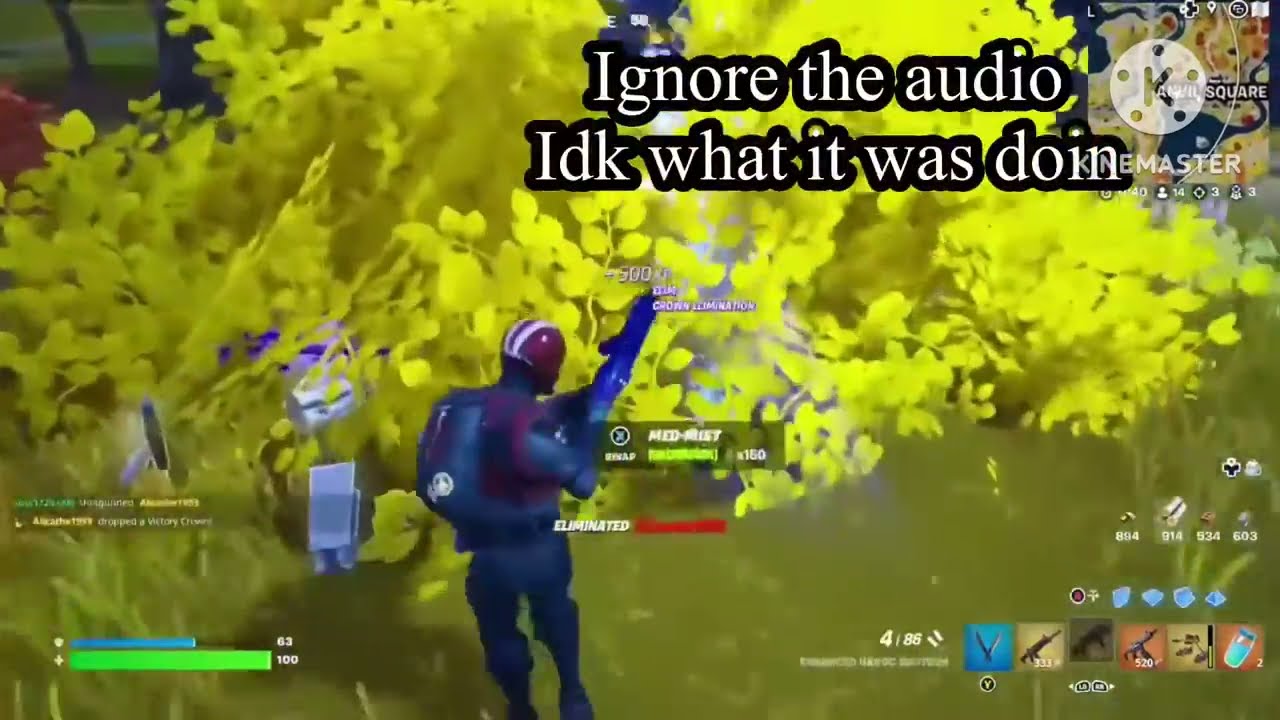This image is a detailed screenshot from a video game, appearing in the middle of a black background with the edges of a screen visible, including a lit-up logo that reads "Vizio" at the bottom. Dominating the scene is a grassy, natural landscape, featuring tall grass in hues of yellow, orange, and green. A character, possibly from Fortnite, is standing or walking through the grassy area; he is wearing a helmet and protective gear that is gray and red, hinting at a military or combat theme. Bordering the grassy field is a river, with additional green patches of grass and numerous rocks on its opposite side. In the distance, a prominent red-leaved tree stands out. 

The upper left corner bears a slightly angled text that reads "like and subscribe" or something similar. Meanwhile, the upper right corner is marked with a watermark from KineMaster, featuring a white circle with a black "K" inside and surrounded by five dots. Additional indistinct text, including "number one victory royale," indicates a win in the game, enhancing the triumphant atmosphere of the screenshot. There are also wood logs or a partial fence visible on the right side, contributing to the scenery's rustic feel.